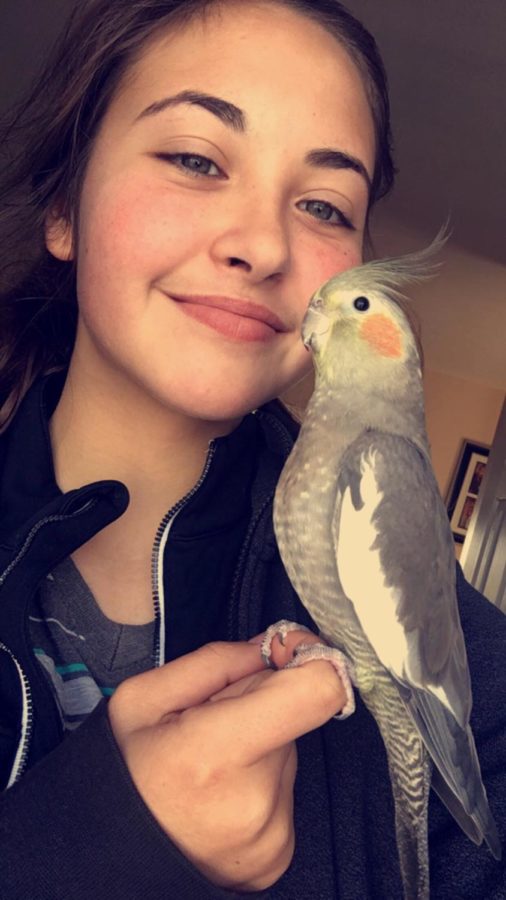The image is a close-up photograph of a young Caucasian teenage girl, smiling warmly at the camera. She has long, dark brown hair loosely pulled back into a ponytail, with just the top of her head slightly cut off in the photo. She is wearing a black sweatshirt with a gray t-shirt underneath. Her right hand is held in front of her chest with her thumb tucked in and pointer finger bent at a 90-degree angle, upon which perches a grey parakeet. The parakeet has distinct features: primarily grey with darker grey wings, a lighter grey chest, white patches on the wings and near its eye, black eyes, orange cheeks, and a tuft of yellow feathers on its head. The photo appears to be taken indoors, likely in a domestic setting, capturing a candid and affectionate moment between the girl and her pet bird.